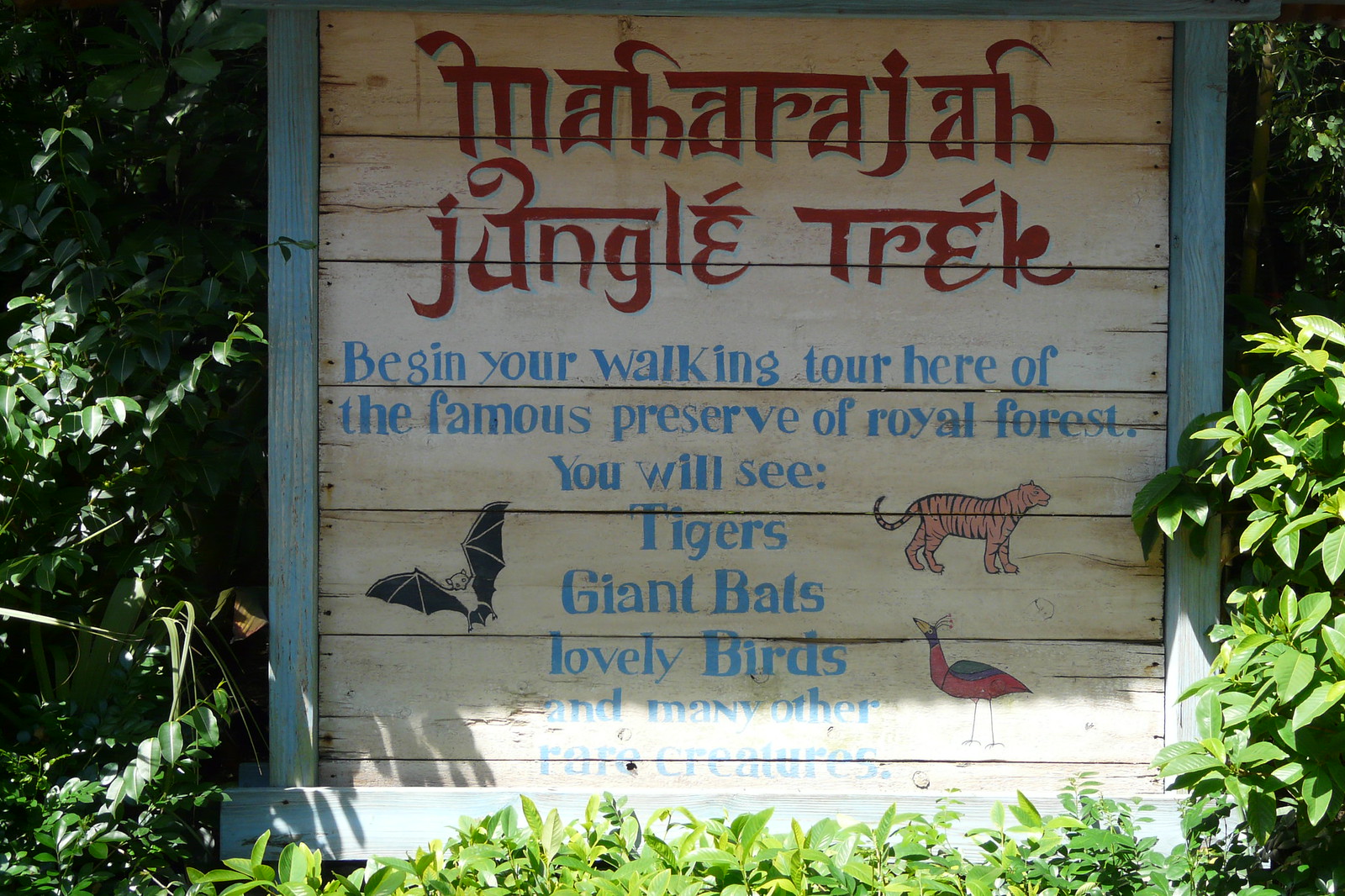The image depicts a large, centrally positioned wooden sign, likely situated within a zoo or nature preserve, amidst dense greenery composed of bushes, trees, and grass. The sign's wood is bordered in light blue, with a series of horizontally oriented planks featuring various elements. At the top, in prominent stylized red lettering, it reads "Maharajah Jungle Trek." Below, blue text invites visitors: "Begin your walking tour here of the famous preserve of Royal Forest. You will see tigers, giant bats, lovely birds, and many other rare creatures." Illustrative graphics of a bat, a tiger, and a bird with thin legs adorn the sign, adding a visual element to the descriptive text. The scene is set outdoors in what appears to be daylight, with the sun casting shadows from the top left. The predominant colors in the image include shades of green, blue, red, and orange, enhancing the natural and inviting ambiance of the scene.